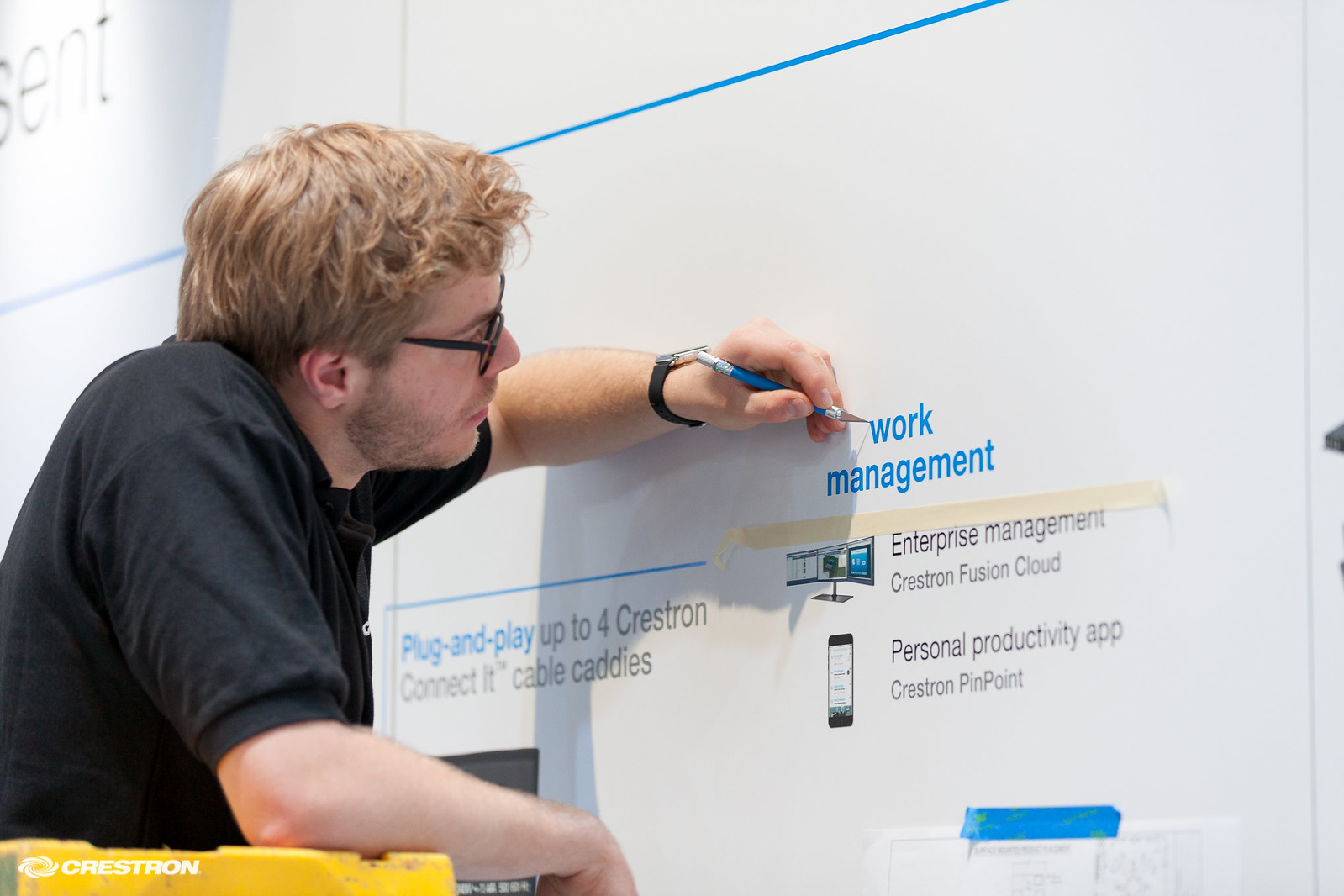This image features a man meticulously working on a whiteboard or poster board during a presentation. At the top of the board, the capital letters "S-E-N-T" are displayed, possibly indicating the company's name. The man, positioned to the right, sports sandy blonde hair, a light beard, and black glasses. He is clad in a black t-shirt and a black wristwatch. His left elbow rests against something yellow, resembling a podium, while he holds a pencil in his right hand, actively writing or editing the content on the board.

The whiteboard prominently features blue lettering, where the phrase "work management" is visible near the top. Below it, there are graphics illustrating "enterprise management," with icons of a computer screen and a phone, adjacent to the term "personal productivity app." The man appears focused and engaged, contributing to what seems to be a detailed and organized presentation on enterprise management and productivity solutions.